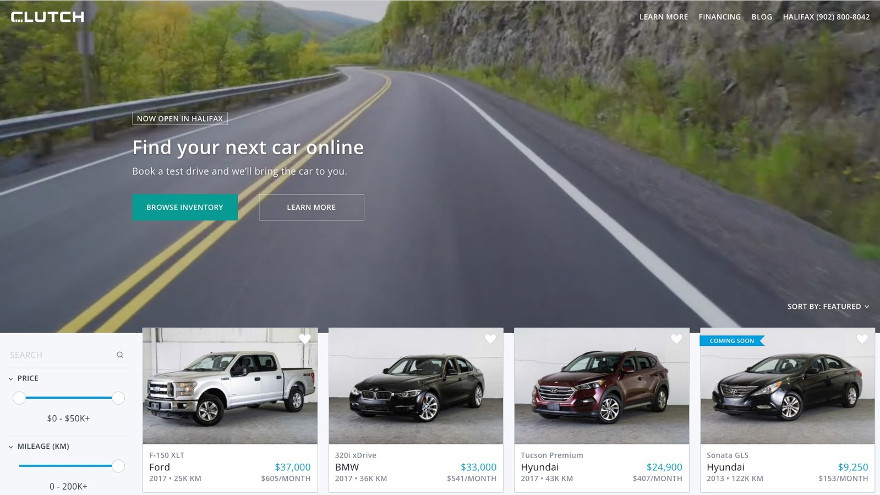A screenshot captures a vehicle sales website named "Clutch," prominently displayed in white text at the upper left corner. In the upper right corner, navigation options include "Learn More," "Financing," and "Blog," alongside a contact number for Halifax: 902-800-8042. Just below, a banner announces, "Now Open in Halifax," with the tagline, "Find your next car online, book a test drive, and we'll bring the car to you.” Two call-to-action buttons — a green "Browse Inventory" and a gray "Learn More" — are positioned beneath this message.

The background features a gray road with a yellow center stripe and a white shoulder stripe, flanked on the left by a metal guardrail and on the right by a rocky cliffside adorned with green and yellow foliage. Descending below, the search parameters allow users to filter cars by price (0 to 50k) and mileage (0 to 200k). Displayed vehicles include:

1. **Ford F-150 XLT** - $37,000
2. **BMW 320i xDrive** - $33,000
3. **Hyundai Tucson Premium** - $24,900
4. **Hyundai Sonata GLS** - $9,250